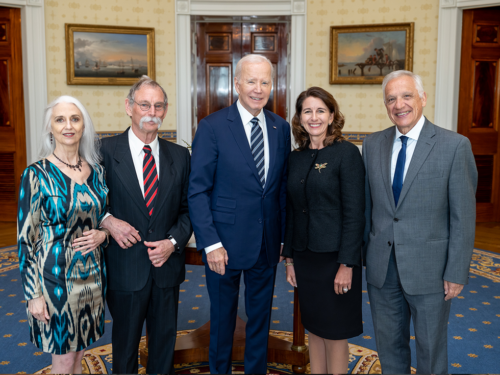In this detailed color photograph of landscape orientation, we see President Joseph Biden standing in the center amid four significant individuals in the Oval Office. From left to right, first is an older woman with long white hair wearing a turquoise blue and beige dress, identified as Robin Friend. Next to her is Joel Siegel, an older man with a long handlebar mustache dressed in a blue suit. President Biden is wearing a light blue suit and standing at the center. To his right is Kathy Warden, CEO of Northrop Grumman, a middle-aged woman with shoulder-length brown hair in a black suit. On the far right stands Janice Yortz, the Dean of USC School of Engineering, an older man with white hair in a gray suit. The background features a blue circular rug, framed historical paintings, wooden doors, and wallpaper of yellow and brown hues. All five individuals are smiling and looking upward in what appears to be an official photo op related to the National Medal for Innovation presentation. The image represents a moment of photographic realism and historical significance.